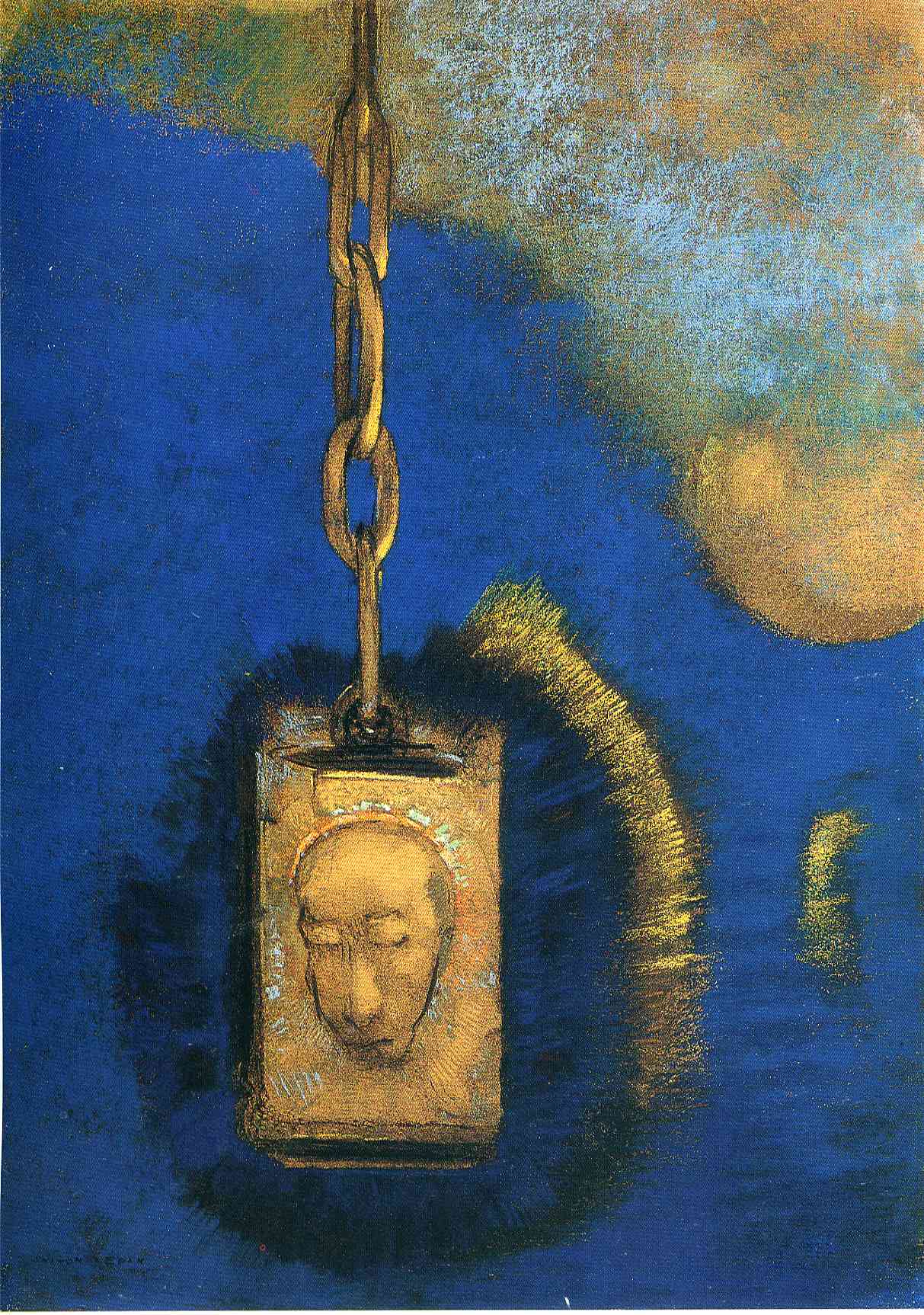This vertically aligned rectangular artwork on canvas features a textured background with a distinct color palette. The top part, especially the upper right section, showcases a blend of brown, gray, and white hues. The rest of the background transitions into various shades of blue, with a majority being a brighter blue interspersed with some darker blue areas. From the top center of the image descends a gold chain, which prominently positions a rectangular gold pendant at its end. The pendant features the outline of a man's head, with closed eyes and a frowning expression. Surrounding the pendant is an aura—a splash of colors including black and a pronounced gold towards the upper right side, forming a circular burst of color. The painting integrates an array of colors, from brown and gray to multiple shades of blue and gold, creating a visually striking piece that feels well-suited for display in a home or museum setting.